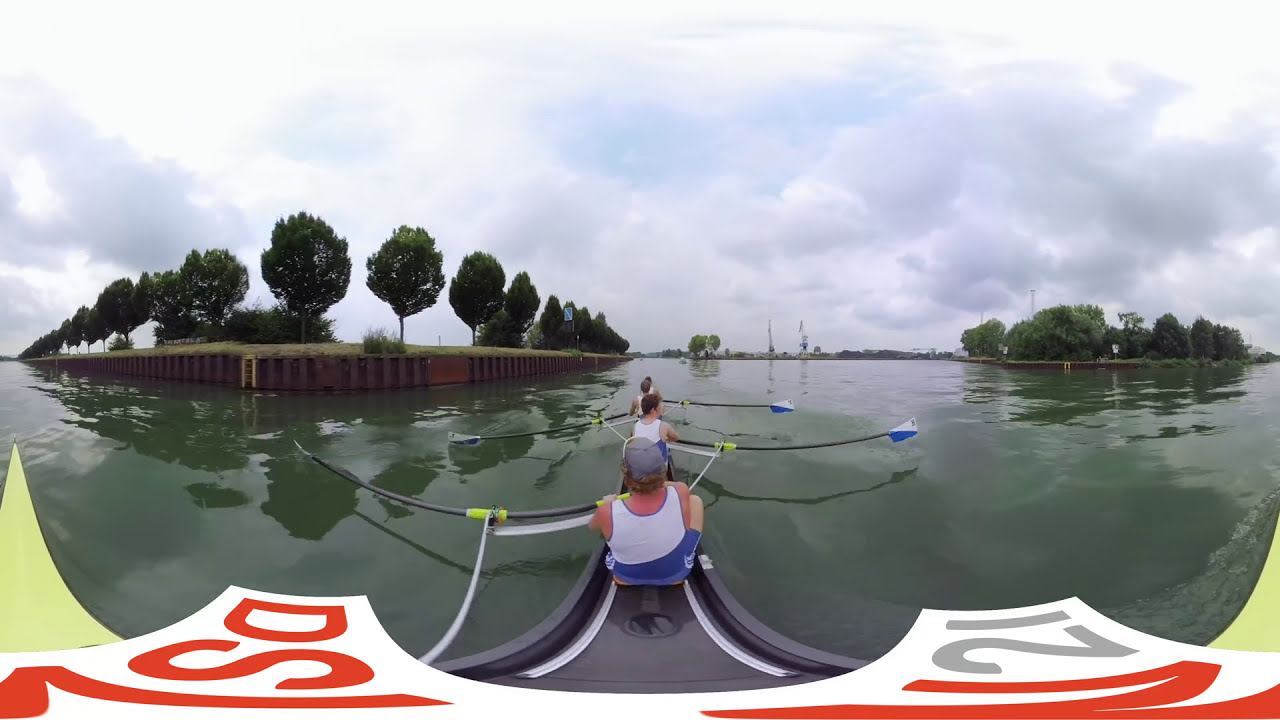This panoramic image, taken from either the front or back of a narrow rowboat, captures three or four individuals actively rowing through a greenish-hued body of water. They all wear white and blue tank tops, and the rower at the back of the boat sports a gray hat. The boat is marked with "N21" on the bottom right side and "DSL" on the bottom left. Four long, gray oars with blue and white striped paddles extend from the boat—two to the right and two to the left.

The water appears reflective, mirroring the surrounding environment, although it is predominantly green. On both sides of the lake, there is a shoreline bordered by rusty metal walls topped with grass and lush green trees. There is also a suggestion of a ladder on the left side, possibly indicating a way out of the water. Above, the sky is dominated by thick, fluffy clouds, leaving little room for blue. Overall, the image has an unusual warped effect along the edges, drawing focus to the rowers centered in the frame.